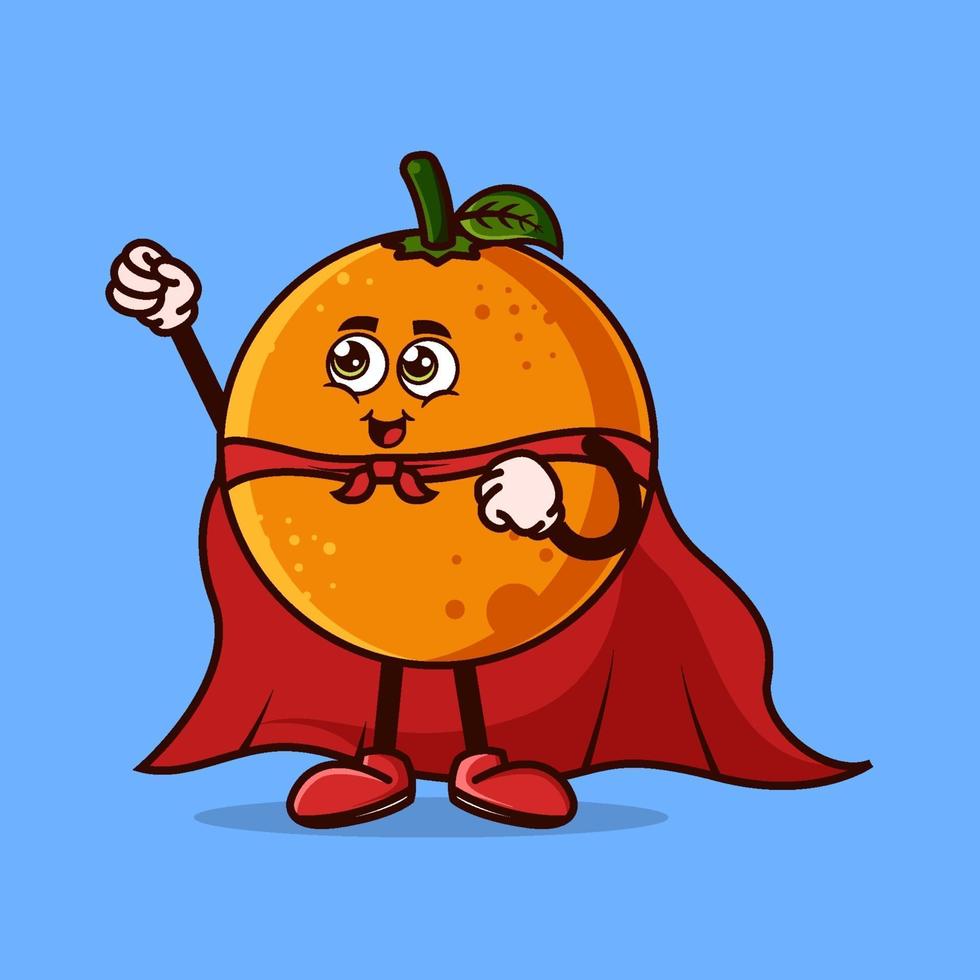This image showcases a digitally-created, cartoon-style orange fruit character set against a sky blue background, embodying a superhero persona. The orange features expressive green eyes, complete with eyebrows and a cheerful smile, giving it a lively and endearing appearance. Sporting a red cape tied around its center, the right hand is enthusiastically raised upward in a classic superhero pose, while the left arm rests closer to its side. Its thin black arms, akin to those of Mickey Mouse, end in white gloved hands. Black-lined legs extend down to red shoes that match the cape, complete with white soles. A small green stem with a single leaf juts out from the top of the orange, adding a whimsical touch. The depiction includes subtle textural details, such as light dots suggesting the orange's surface and light shading to indicate a light source from the left, enhancing the three-dimensional feel of the character.